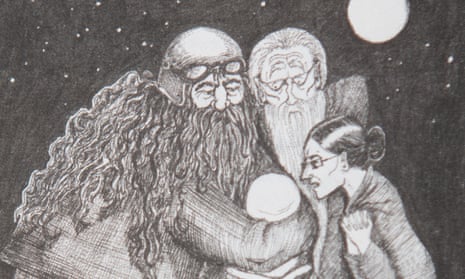This black-and-white hand-drawn sketch, an early concept by J.K. Rowling for "Harry Potter and the Philosopher's Stone," depicts three key characters in a night setting. Positioned beneath a starry sky with a full moon in the top right, a bulky bearded man on the left, likely Hagrid, dons a helmet with goggles atop his head. His long hair and beard flow down to his chest. Hagrid's gentle gaze is focused on what he cradles in his arms—probably a baby, presumably Harry Potter. Next to him stands an elderly man with long white hair, a matching beard, and wire-framed glasses, reminiscent of a Merlin-like figure. Beside him, a stern-looking woman with dark hair pulled into a bun, also wearing glasses, observes intently. All three characters are transfixed by the baby in Hagrid's arms, suggesting they play crucial roles in the infant's future. The grainy texture of the image implies it might have been photographed, adding a sense of authenticity to this early artistic vision.